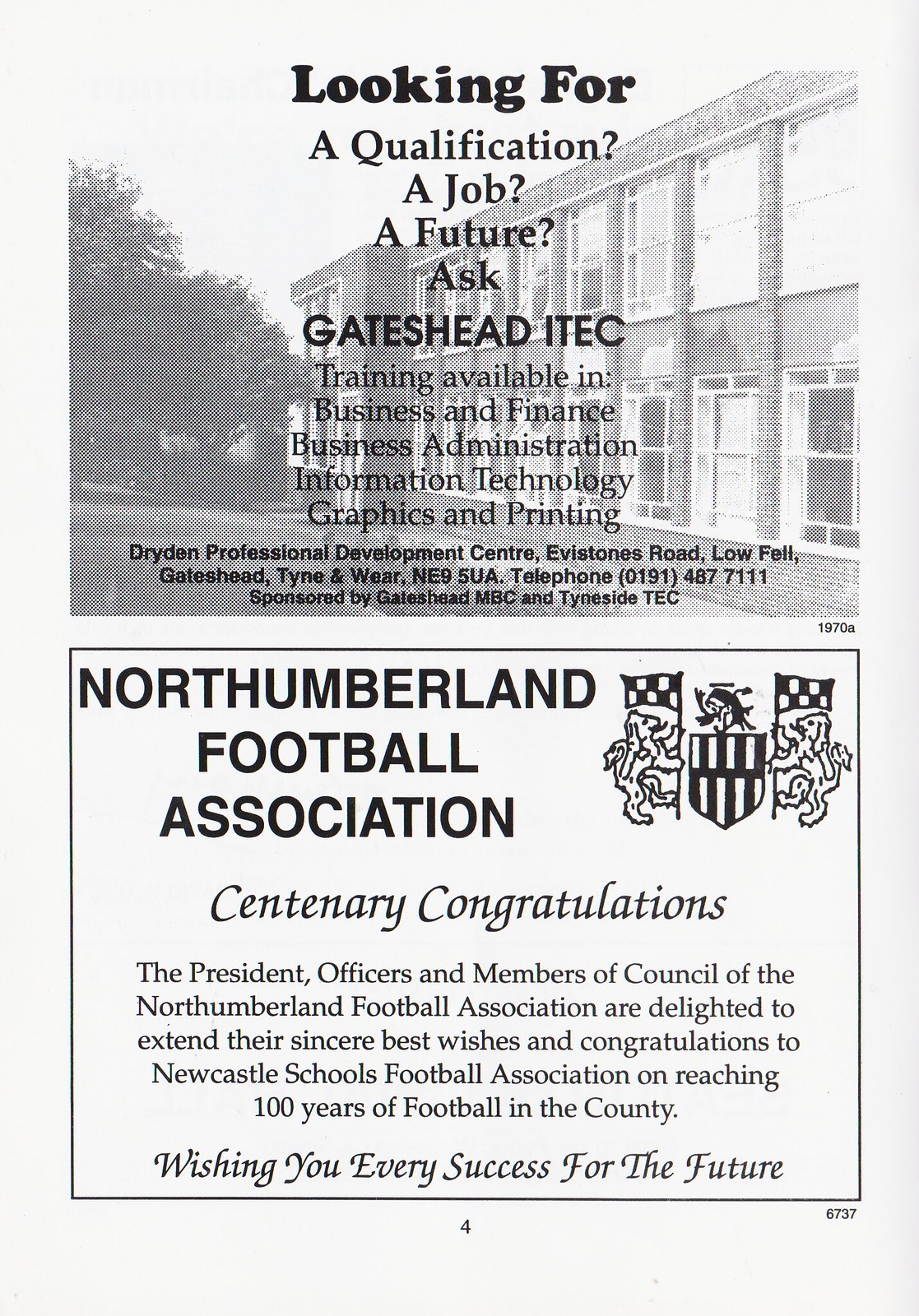The image displays two distinct sections featuring business and celebratory content. The top portion is an advertisement from Gateshead ITEC, encouraging individuals to seek qualifications, jobs, and futures through training available in business and finance, business administration, information technology, graphics, and printing. The ad provides the contact information: Dryden Professional Development Center, Evaston Road, Lofell, Gateshead, Tyne and Wear, NE9EUA, telephone 0191-4877-1111. This section is sponsored by Gateshead MVC and Tideside TEC and includes a dotted illustration of a building in the background. Below this, there is a congratulatory message from the Northumberland Football Association. The message, adorned with a logo depicting two lions holding flags and a shield, extends sincere best wishes to the Newcastle Schools Football Association on their centenary, celebrating 100 years of football in the county. Additionally, the page is marked with the number four in the middle and the numerical sequence 6737 at the bottom right.